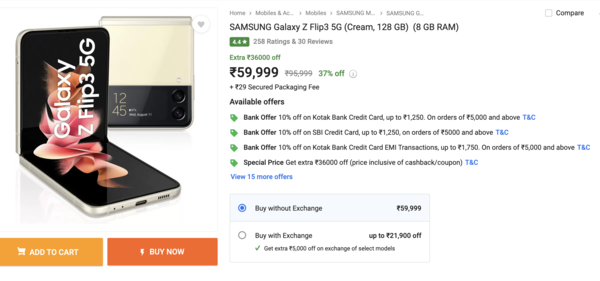Screenshot of a Samsung Galaxy Z Flip 3 5G for Sale:

The image captures a detailed online listing for a Samsung Galaxy Z Flip 3 5G, which is being sold in the color "Cream." Technical specifications include 128GB of internal storage and 8GB of RAM. The device has an overall rating of 4.4 stars from 258 reviewers, accumulated through 30 individual reviews.

The price shown is 37% off from its initial amount, reducing from 59,999 to 36,000 in an unspecified currency, with a secure packaging fee included. Payment options are mentioned, including several bank offers: 
- 10% off on Kodak Bank credit card transactions up to 1,250 on orders over 5,000
- 10% off on SBI credit card transactions up to 1,250 on orders over 5,000
- 10% off on Kodak Bank credit card EMI transactions

A special price promotion provides an extra discount of 36,000. The device is available with or without exchange, with up to 21,900 off for device exchanges and an additional 5,000 off for select model exchanges.

Controls to "Add to Cart," "Buy Now," and "Compare" are provided on the screen. The visual includes two images of the Galaxy Z Flip 3: one showing the phone open and another showing the phone closed.